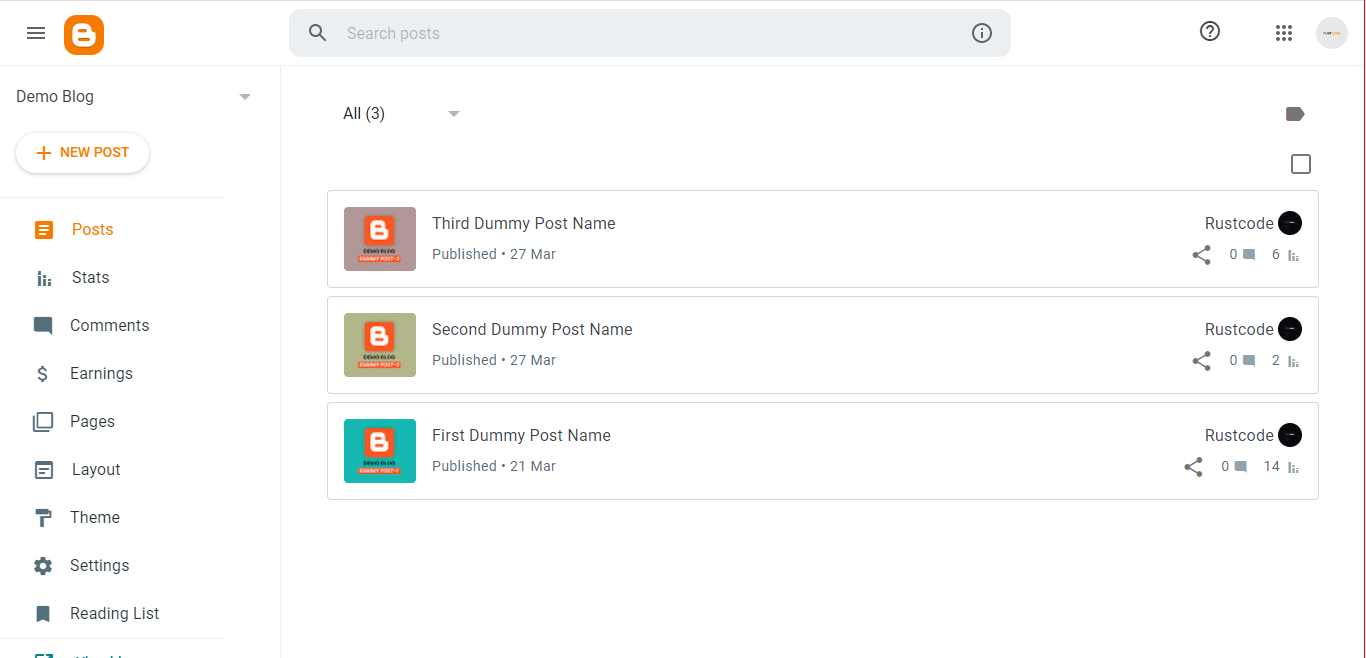The image depicts a website interface showcasing a blog management service. At the top center of the page is a prominent search box. On the left sidebar, there are various navigational options listed: "Demo Blog," "New Posts," "Posts," "Stats," "Comments," "Earnings," "Pages," "Layout," "Theme," "Settings," and "Reading Lists."

In the main content area, a section titled "All," followed by the number 3 in parentheses, indicates the count of posts available. Below this, there are three blog post entries listed chronologically:
1. "Third Dummy Post Name," published on March 27th.
2. "Second Dummy Post Name," published on March 27th.
3. "First Dummy Post Name," published on March 21st.

To the right of each post entry, there is an icon of a black circle with the label "Rust Code."